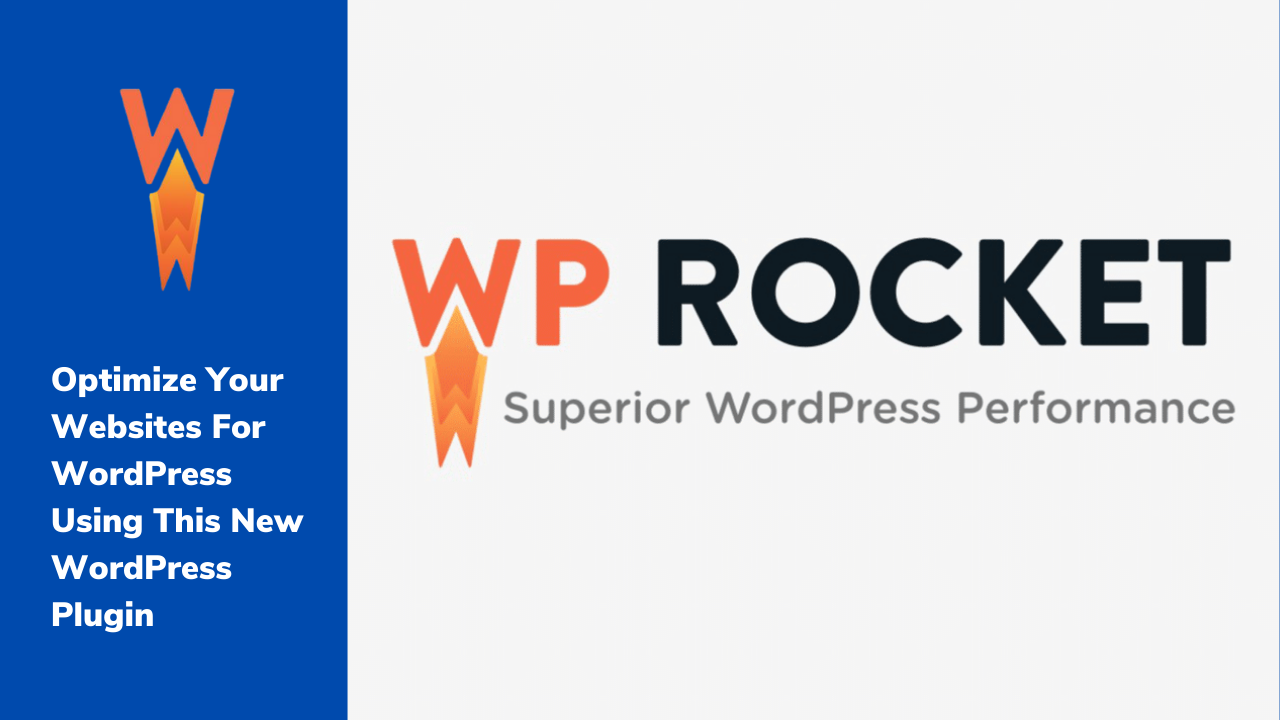The image is the front page of a website, featuring a two-color background. On the left side, there is a broad vertical stripe in royal blue. This stripe showcases an orange "W" with flames emerging from the bottom, creating a dynamic visual effect. The text on this blue section reads: "Optimize your websites for WordPress using this new WordPress plugin," written in a bold, impactful font.

The rest of the page has a clean white background. Positioned prominently on this white section are the letters "WP," with the "W" in orange—complete with flames, similar to those on the blue stripe—and the "P" in orange as well. Below these letters, the bold, black, all-caps text reads: "WP ROCKET," standing out in thick, robust lettering. Beneath this, in an upper and lower case gray font, the tagline states: "Superior WordPress Performance."

There are three distinct fonts used on the page: a powerful one for "WP ROCKET," a less striking gray font for the subtitle, and a strong, bold font for the text on the blue stripe, emphasizing the plugin's benefits.